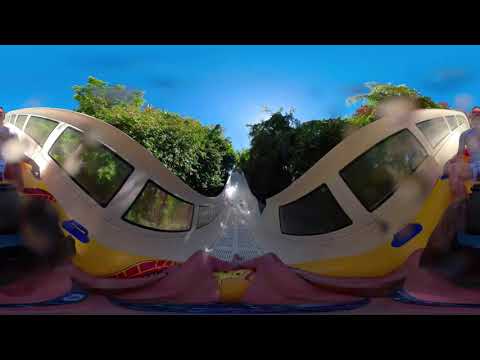This image is a small rectangular photograph with thick black borders at the top and bottom, depicting a highly distorted view that appears to be taken with a 360-degree camera lens. The central focus of the image presents an abstract, almost bra-shaped white object, adorned with windows—five on each side—resembling a train or vehicle's compartments. This white object has a yellow section at its base, transitioning into a pink area that seems to touch the surface below. Flanking the object on both sides are varying shades of green trees and bushes, with a very blue, cloudless sky above them. The bright sun peeks through the foliage, contributing to the high-contrast, vivid atmosphere of the scene.